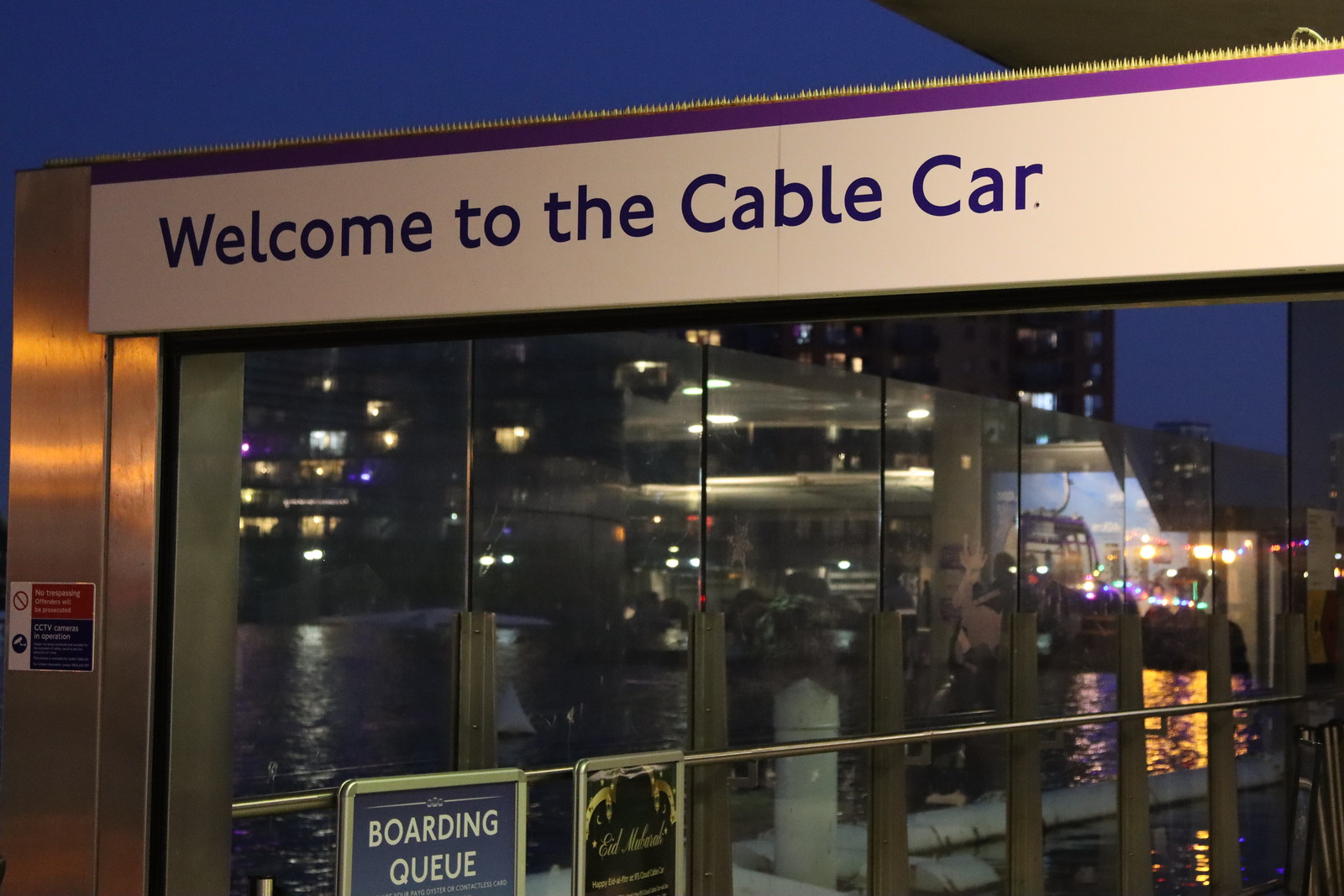This horizontal-rectangular nighttime photograph showcases the entrance to a cable car system. Dominating the top of the image is a prominent sign that reads "Welcome to the Cable Car," set against a deep blue sky. Beneath the sign, a metallic gateway flanked by reflective surfaces hints at an urban landscape, with mirrors revealing the reflections of surrounding buildings and a body of water. Bright orange lights punctuate the scene on the left, casting glows onto the reflective metals and adding warmth to the cool night tones.

A fenced pathway guides prospective passengers, with signs clearly marking the "Boarding Queue." These signs are attached to a metallic railing that extends across the image, steering the flow of people towards the entrance. The building in the background, not fully visible but heavily illuminated, adds a bustling ambiance to the setting. Warning posters and various boards with designs add to the visual interest, creating a detailed snapshot that captures the organized albeit vibrant atmosphere of the cable car boarding area at night.